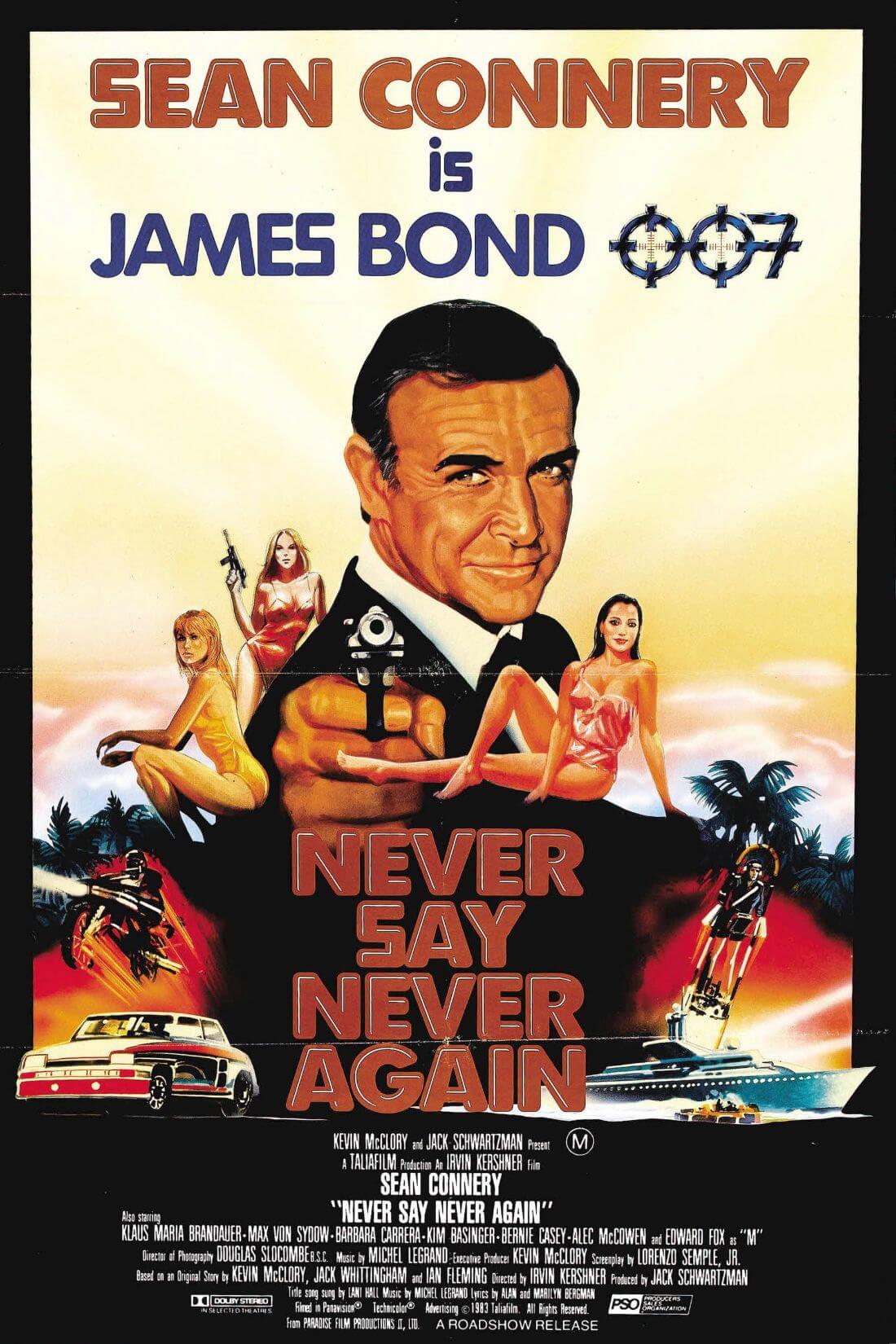The movie poster for "Never Say Never Again" features a young, handsome Sean Connery as James Bond 007, with a broad, smug smile, pointing a black gun directly at the viewer. The design has an old-school, pulp fiction flair with a vibrant, yellowish sky background. The layout is vertically oriented within a black border, with the title "Never Say Never Again" written on Bond's suit in striking red font. Surrounding Bond are three women dressed in swimsuits: one lounging on the ground, another crouching, and a third standing confidently behind him, holding an Uzi or machine gun.

Additional dynamic elements populate the poster, including a muscle car in the bottom left corner, an airborne motorcycle above it, and a speedboat in the bottom right corner. Palm trees add a touch of tropical flair to the chaotic action depicted. Text details in various colors—"Sean Connery" in red, "is James Bond" in blue, and "007" with zeroes as rifle crosshairs—cascade down the top of the poster. Beneath the main illustration, a black text box provides further credits and details about the movie.